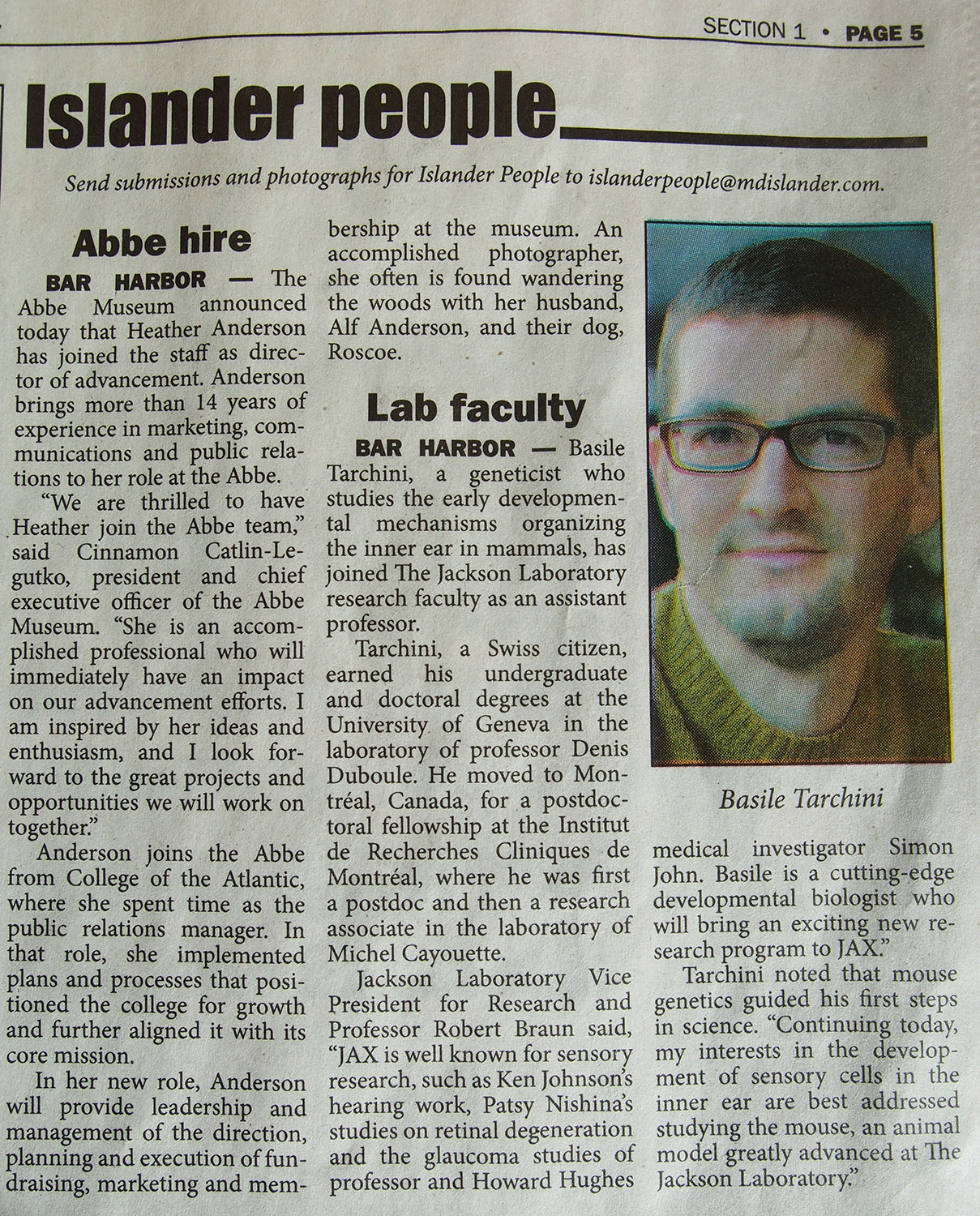In the newspaper's Section 1, Page 5, there is an article featuring two significant updates in the Bar Harbor community. The piece highlights the announcement from Abbey Museum regarding the appointment of Heather Anderson as the Director of Advancement. With more than 14 years of experience in marketing, communication, and public relations, Anderson is expected to bring considerable expertise to her new role. 

Additionally, the article introduces Basil Taccini, a new faculty member at Jackson Laboratory. Taccini, a geneticist specializing in the early developmental mechanisms of the inner ear in mammals, has joined the research faculty as an assistant professor. A Swiss citizen, Taccini completed both his undergraduate and doctoral studies at the University of Geneva. 

The accompanying photograph shows Basil Taccini, who has a fair complexion, short brown hair, black glasses, and a 5 o'clock shadow.

For further information or to send submissions and photographs for the Islander people section, readers are encouraged to contact islanderpeople@mdislander.com.